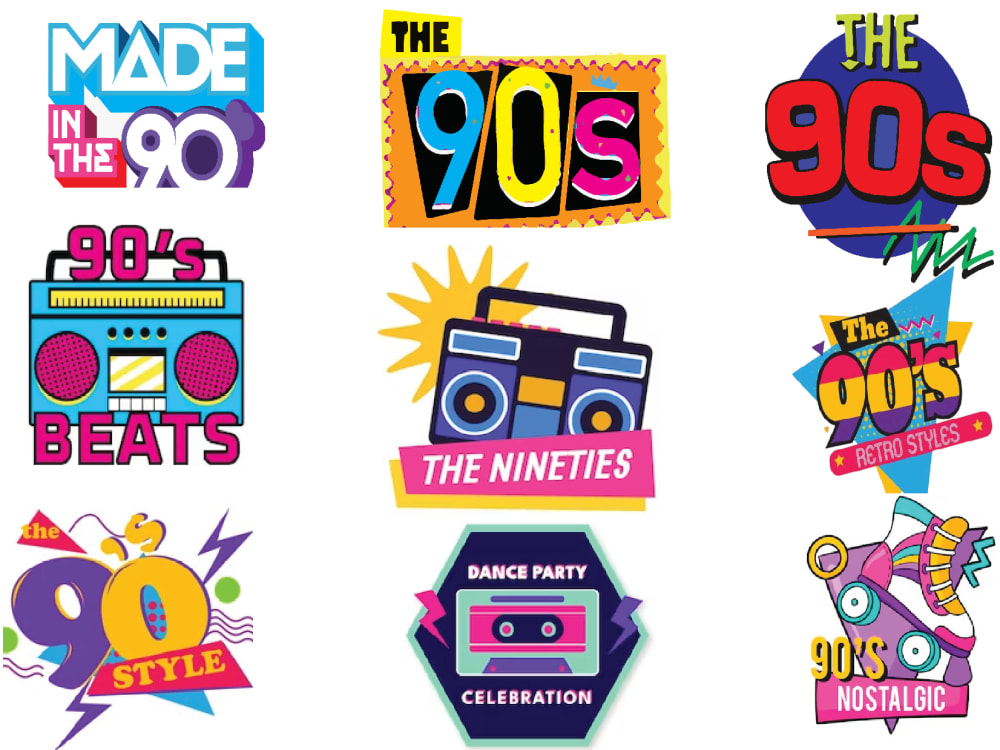This image comprises nine vibrant, sticker-like icons presented in a landscape orientation, all centered around 1990s music and culture. Each icon showcases unique 90s-themed designs and bright colors against a clean, white background.

1. **Top Left Corner**: Features "Made in the 90s" in three-dimensional block letters. "Made" is rendered in white with a blue outline, while "in the" appears in white letters on a pink and purple block. The "90s" is large, white, and outlined in purple.
   
2. **Top Center**: Resembles a postage stamp with "the" in black letters on a yellow background, enclosed in an orange box with grooved edges. The "90s" is split into a blue '9' on a black background, a yellow '0' on a black background, and a pink 'S.'

3. **Top Right Corner**: Displays "the 90s" in yellow and red, set against a purple circle. Squiggly lines embellish the bottom of the design, adding a playful touch.

4. **Middle Left**: Portrays a blue radio with pink speakers and white cassette player buttons, captioned "90s Beats" in pink.

5. **Center**: Features another radio, this time in purple, against a sunburst design. Below, it says "the 90s" in pink and yellow.

6. **Middle Right**: Contains parallelogram and triangular shapes in blue and yellow, with the label "the 90s retro styles" in pink, purple, and yellow.

7. **Bottom Left**: Depicts "the 90s style" in white on a pink triangle, with "style" in a pink box. The '9' is purple and the '0' is yellow.

8. **Bottom Center**: Shows a teal and pink cassette tape within a dark blue hexagon with a teal border. Surrounding this, "Dance Party Celebration" is written in white letters.

9. **Bottom Right Corner**: Contains a purple triangle backdrop with zigzags and circles, featuring a roller skate with a rainbow and teal wheels. Below it, "90s" is written in yellow, followed by "Nostalgic" in white letters inside a pink box.

The cohesive theme and lively colors emphasize the nostalgic feel of the 90s music era across all nine designs.